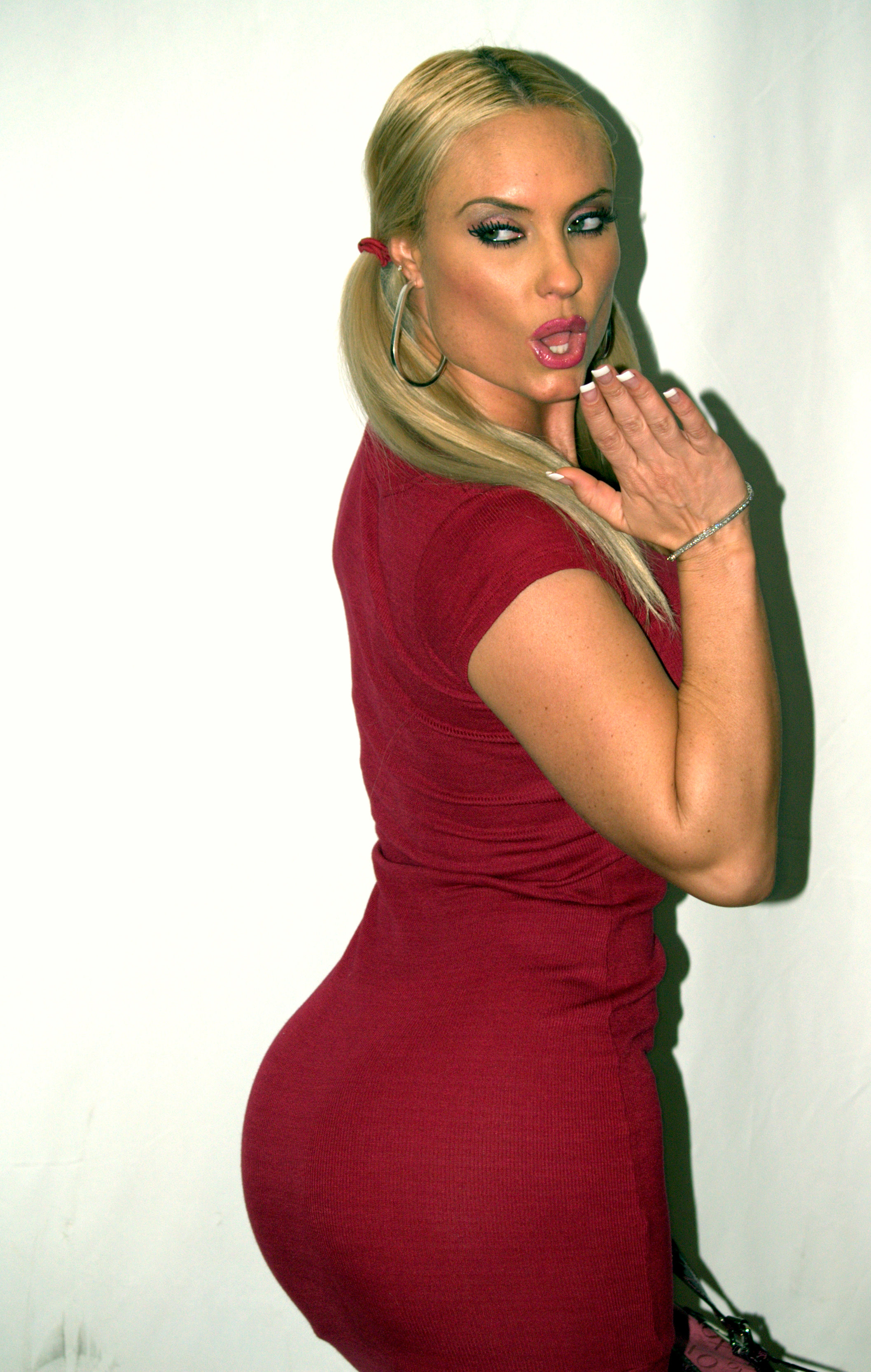The photograph depicts a middle-aged blonde woman with her hair styled in pigtails, posing with her back partially facing the camera while turning around to blow a kiss. She is dressed in a vibrant raspberry-colored dress and has heavy makeup on. Her nails are painted with a mix of white and black polish. A small bracelet adorns her right wrist. The setting is brightly lit with natural light, showcasing a clear view free of any other people, text, or numbers. The background appears to be a plain white wall. Her cheerful and whimsical demeanor contrasts with her mature age, creating a unique and eye-catching image.